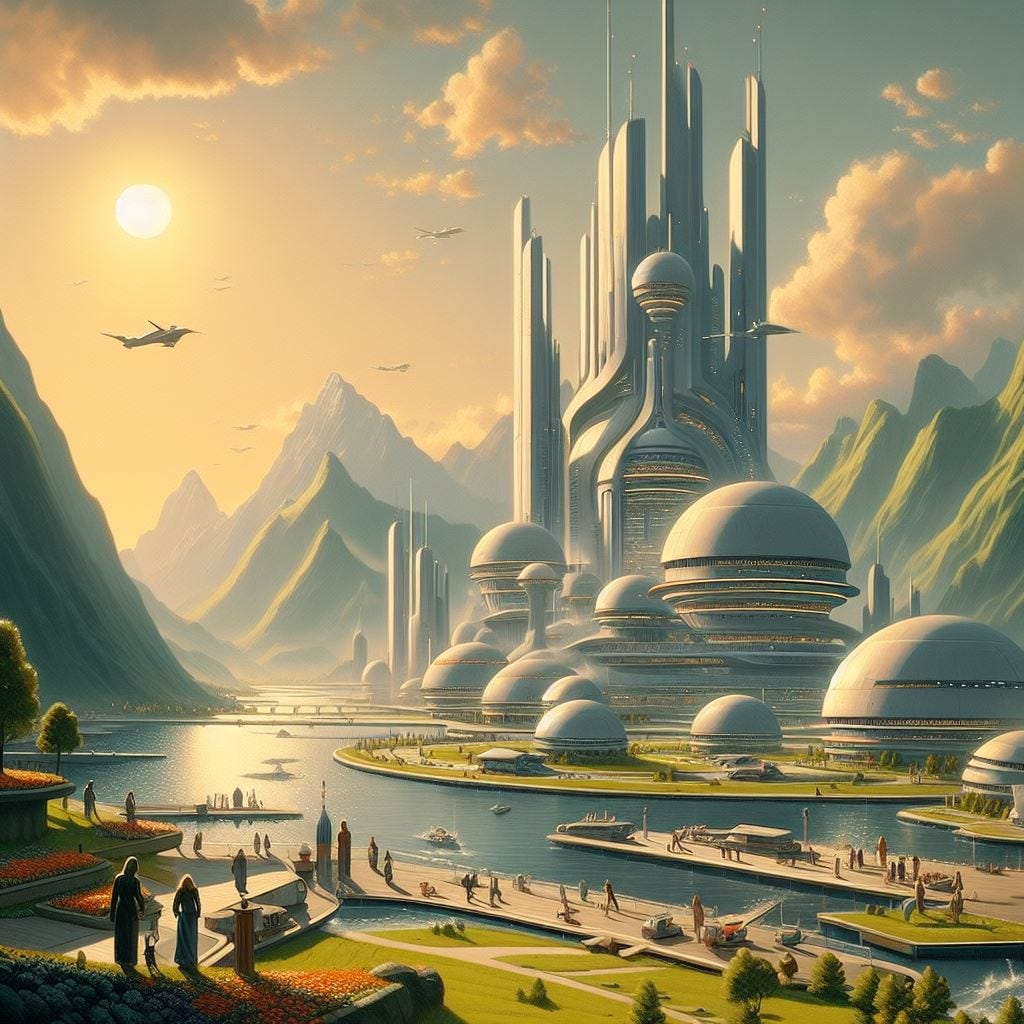In this digital artwork depicting a futuristic or otherworldly cityscape, we observe a vibrant, circular city emerging from a lush, mountainous valley. The city is a blend of half-spherical domes and towering skyscrapers, encircled by a public garden and a park teeming with greenery. The scene is set during the twilight with a setting sun casting its glow, creating a spectrum of colors including grays, greens, reds, and yellows. In the sky, various aircraft glide, with one plane prominently in the foreground and three more in the hazy distance, all flying eastward. People are scattered around, engaging with the serene garden area, adding to the utopian feel of the place. Additionally, water bodies with boats suggest a waterfront setting, reminiscent of a port city nestled amidst the mountains. The artwork's surreal and detailed portrayal gives it a unique, almost 3D visual effect, capturing the essence of a harmonious futuristic world.